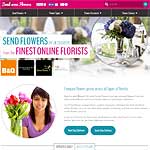The screenshot captures a section of a flower delivery website. The image is rectangular and prominently features a bright hot pink bar running across the top. Within this bar, white text displays various navigational options for the site. On the right side of this bar, there's a darker pink search bar.

Beneath this, an area is highlighted with information about the website in bright blue text on a white background, reading "Send Flowers". Below this, in hot pink text, the tagline "Finest Ornate Florists" is displayed.

The background features somewhat blurry images of flowers, predominantly dark blue with hints of green foliage, making them difficult to distinguish clearly. Below this background, a circular inset displays an image of a woman with medium-length black hair and bangs, wearing a purple V-neck shirt. The woman is positioned next to a large bouquet of pink flowers with green stems, which are tied in the middle.

The background of the entire scene is white. Additional elements include various buttons and links in gray, blue, and turquoise, with the turquoise buttons having white text on them.